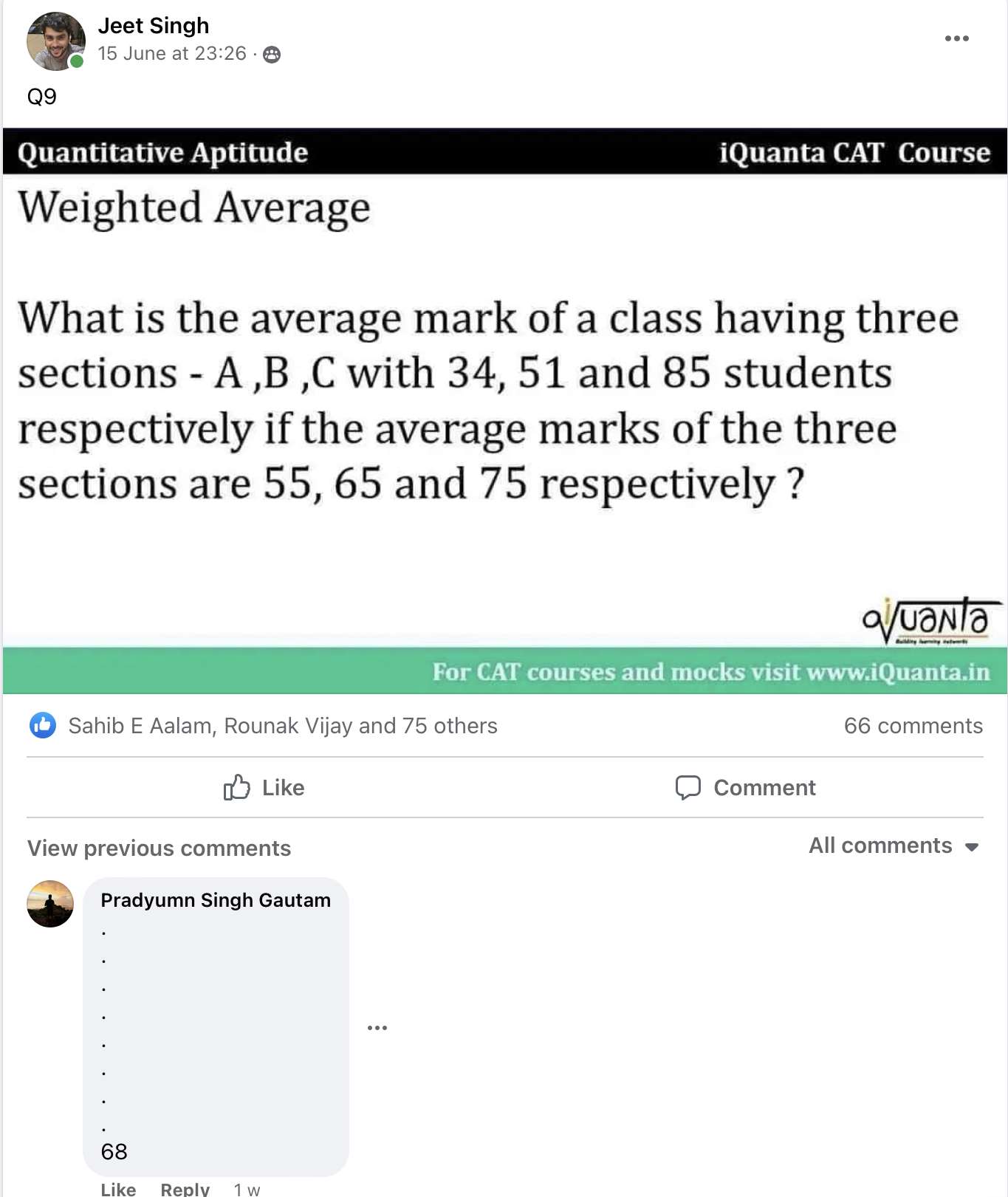The image displays a comprehensive scene regarding a Quantitative Aptitude topic, particularly focusing on a weighted average problem. 

In the top left corner of the image, there is a section listing names such as Jeet Singh and Bhutan Juran, along with numbers 23, 26, and 29. This part implies a segmentation likely related to viewing options or timestamps. Below this, the text "Quantitative Aptitude" is clearly marked followed by an "Icon.cat course," suggesting an educational module or lesson from the iQuanta platform.

The primary focus of the image involves a math problem statement: "What is the average mark of a class having three sections, A, B, and C, with 34, 51, and 85 students, respectively, if the average marks of the three sections are 5, 6, and 7, respectively?" This is prominently displayed to highlight the subject of the example being explained.

Additionally, there is a promotional banner stating, "For CAT courses and marks, visit www.iQuanta.in," accompanied by the iQuanta logo.

The bottom portion of the image consists of a social media interface where it shows interaction details: the post has received likes from users, including Sahib, E, Alan, Brunek, Vijay, and 75 others, alongside 3 to 6 comments, thumbs up, comment buttons, and a preview text indicating previous and all comments. 

An image of Pradyum, Sindh, Bhutan is referenced, alongside the number 68 and a label indicating "like," "reply," and "one week" markings—likely to represent the engagement metrics of the post.

Finally, there is a mention of "Q9 something shared a social media post," indicating that it has been re-shared, and someone posting their answer to the problem, marked as "68."